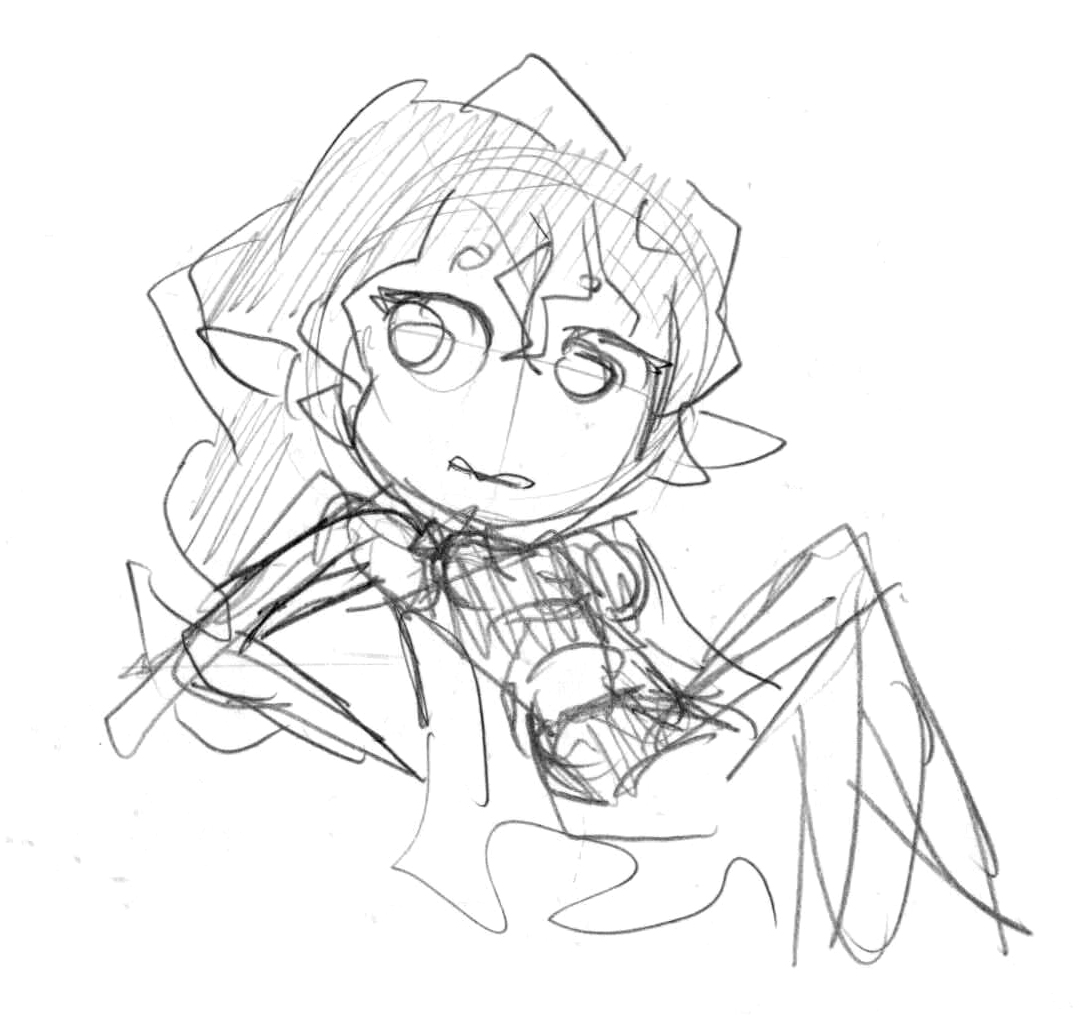The image depicts a very crude, rough pencil sketch of a young female anime-style cartoon character. The figure is characterized by extremely large, hollow eyes and an oversized head, approximately three times the width of her torso, giving her a distinctive, exaggerated appearance. Her long hair is represented by simple scribbles without any shading. She seems to be wearing a cropped top, though the details are minimally defined. The drawing lacks intricate features, employing just basic lines for her limbs, with no detailed bends or hands. The character is propped up on her right arm while reclining with her legs bent at a 90-degree angle. She is looking directly at the viewer, though her gaze lacks detail. The entire sketch is monochromatic, executed hastily with a regular lead pencil, embodying a very rudimentary and simplistic style.